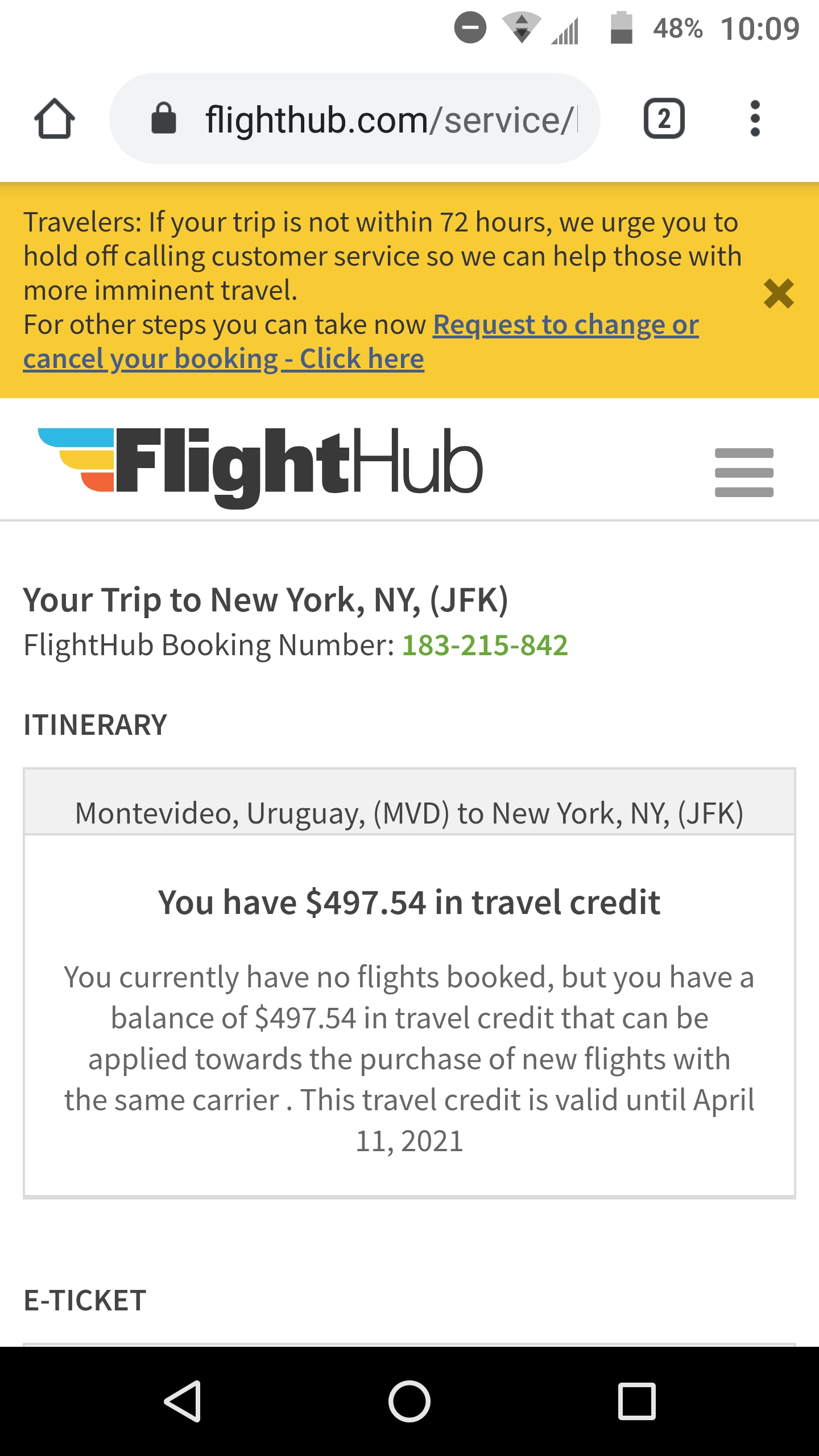### Screenshot Description:

The screenshot captures a webpage from FlightHub.com as displayed on a smartphone. At the top of the screen, various icons and indicators are visible, including a dark circle with a white dash, a Wi-Fi signal icon with up and down arrows, full carrier signal bars, and a battery indicator showing 48% battery life. The current time displayed is 10:09 AM. The phone's home button is visible at the bottom of the screen.

#### Website Header and Navigation:
- **FlightHub.com URL**: The URL bar shows "flighthub.com" with a secure lock icon indicating the connection is secure. 
- **Tab Indicator**: The number "2" in a square indicates two open tabs.
- **Options Menu**: A three-dot menu for additional options.
- **Alert Banner**: A yellow rectangle with the message, "Travelers: If your trip is not within 72 hours, we urge you to hold off calling customer service so we can help those with more imminent travel. For other steps you can take now, [request to change or cancel your booking - click here]."

### Website Branding:
- **Logo**: "Flight" in bold, "hub" in regular font next to the logo featuring three diagonal bars in blue, yellow, and red.

### Main Content:
- **Header Text**: "Your trip to New York, New York (JFK)"
- **Booking Number**: FlightHub booking number: 183-215-842 (green text).
- **Section Title**: "ITINERARY" in capital letters.

#### Itinerary Details:
- **Travel Route**: Montevideo, Uruguay (MVD) to New York, New York (JFK).
- **Travel Credit Notice**: 
  - Bold Text: "$497.54 in travel credit"
  - Message: "You currently have no flights booked but you have a balance of $497.54 in travel credit that can be applied towards the purchase of new flights with the same carrier. This travel credit is valid until April 11th, 2021."
- **E-Ticket**: Label "e-ticket" appears below the credit notice.

### Footer Navigation:
- A black bar at the bottom of the phone screen containing navigation icons: a white arrow, a white circle, and a white square.

The overall layout of the screenshot includes user-friendly alerts, navigation options to manage bookings, and a detailed display of available travel credits.